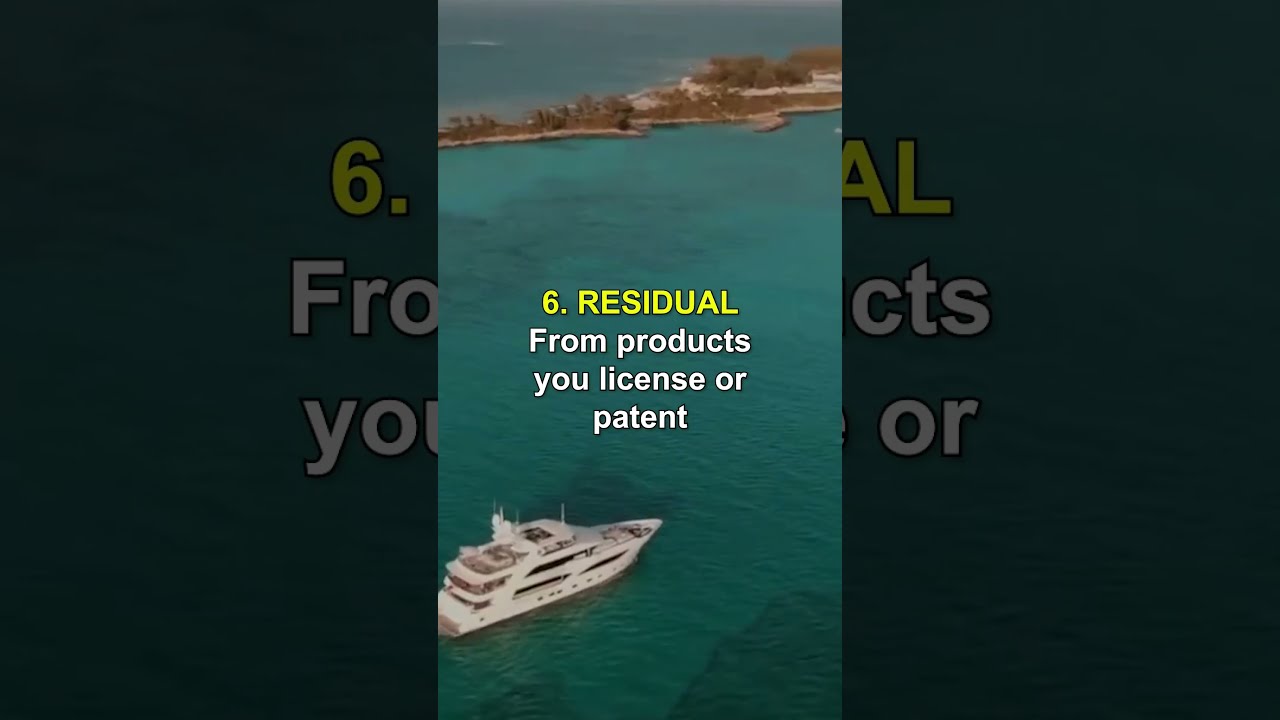This image appears to be a frame from a video, as indicated by the caption "6 PERIOD RESIDUAL from products, you license or patent," with "6 PERIOD RESIDUAL" in yellow text and the rest in white. The scene is an overhead, drone-like shot featuring a turquoise, transparent ocean in which a three-story, white luxury yacht with black windows is positioned in the bottom left corner. Above, towards the top, there's a small strip of land that resembles a sandbar with trees and vegetation, and possibly some form of land structure or port, though the resolution makes it difficult to discern. The overall shape of the image is similar to that of a high-definition TV, bordered on the sides by black with the central photograph maintaining a vertical, cell phone-like format. This likely represents part of a visual presentation in a financial advice video, emphasizing residual income from licensed or patented products.